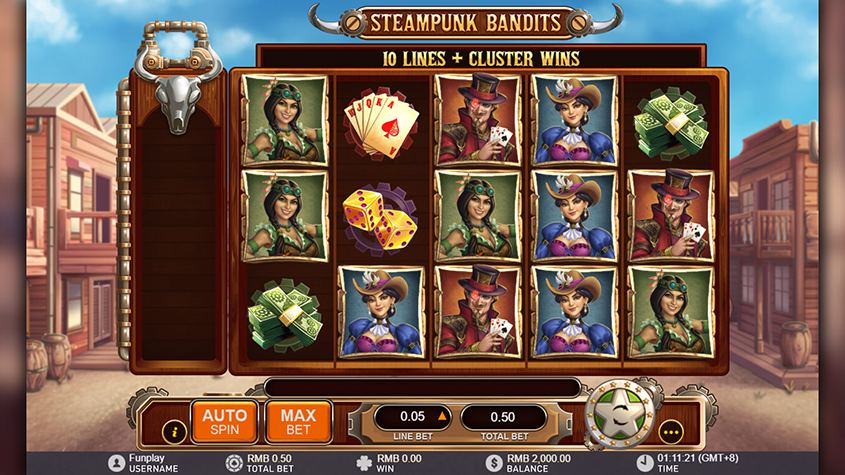The front page of this video game features a title at the top that reads "Steampunk Bandits." Below the title, text highlights gameplay elements such as "Ten Lines Plus Cluster Wins." The interface resembles a large bulletin board with numerous listed characters, many of whom are shown multiple times. Scattered across the board are various game elements including cards, a pile of dice, and two piles of money. Instructions for game functions like "Auto Spin," "Max Bet," "Line Bet," "Total Bet," indicate that this is a betting game. The background depicts an Old Western scene with a dirt ground and wooden houses with wooden porches and sidewalks lining the street. At the very bottom of the screen, essential player information such as username, total bet, win amount, balance, and the current time is displayed.